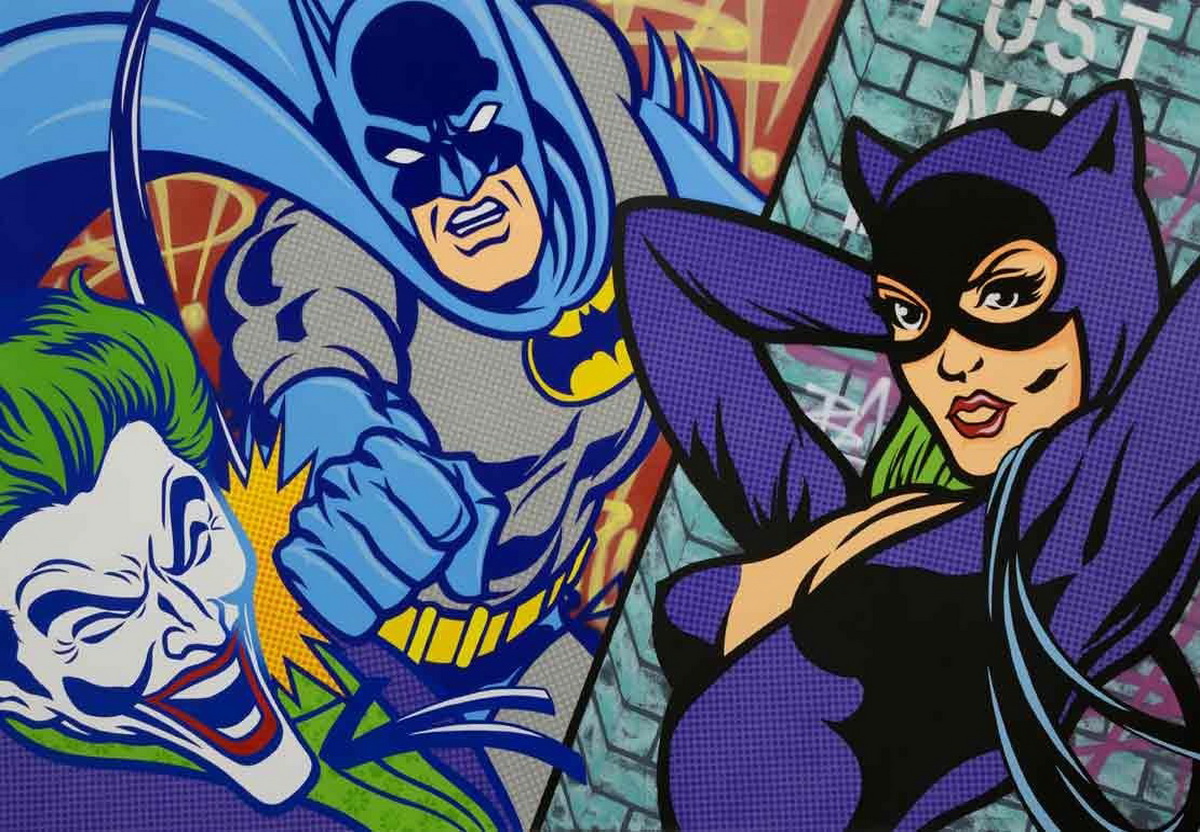The image is a detailed comic book scene featuring Batman, the Joker, and Catwoman. Batman, centrally positioned, is delivering a punch to the Joker's face. Batman is depicted with a mean expression, wearing a blue cape, a gray bodysuit with a yellow and black bat symbol, blue gloves, and a yellow utility belt. His right fist is connecting with the Joker's face, creating an explosion mark on impact. The Joker, located in the lower left side, has green hair, a big smile with red lipstick, and white clown makeup. He is reeling from the punch, squinting in pain, with his head turned to the side.

To the right of Batman stands Catwoman against a background of greenish-blue bricks with some white graffiti letters visible. Catwoman is in a provocative purple bodysuit with chest exposure, accessorized with black gloves, a black face mask, and purple cat ears. She has long black hair, red lipstick, and a seductive smile. Catwoman's hands are posed behind her head, adding to her alluring stance. The backgrounds for Batman and the Joker feature reddish-yellow hues, providing a stark contrast to Catwoman's bluish-brick setting.